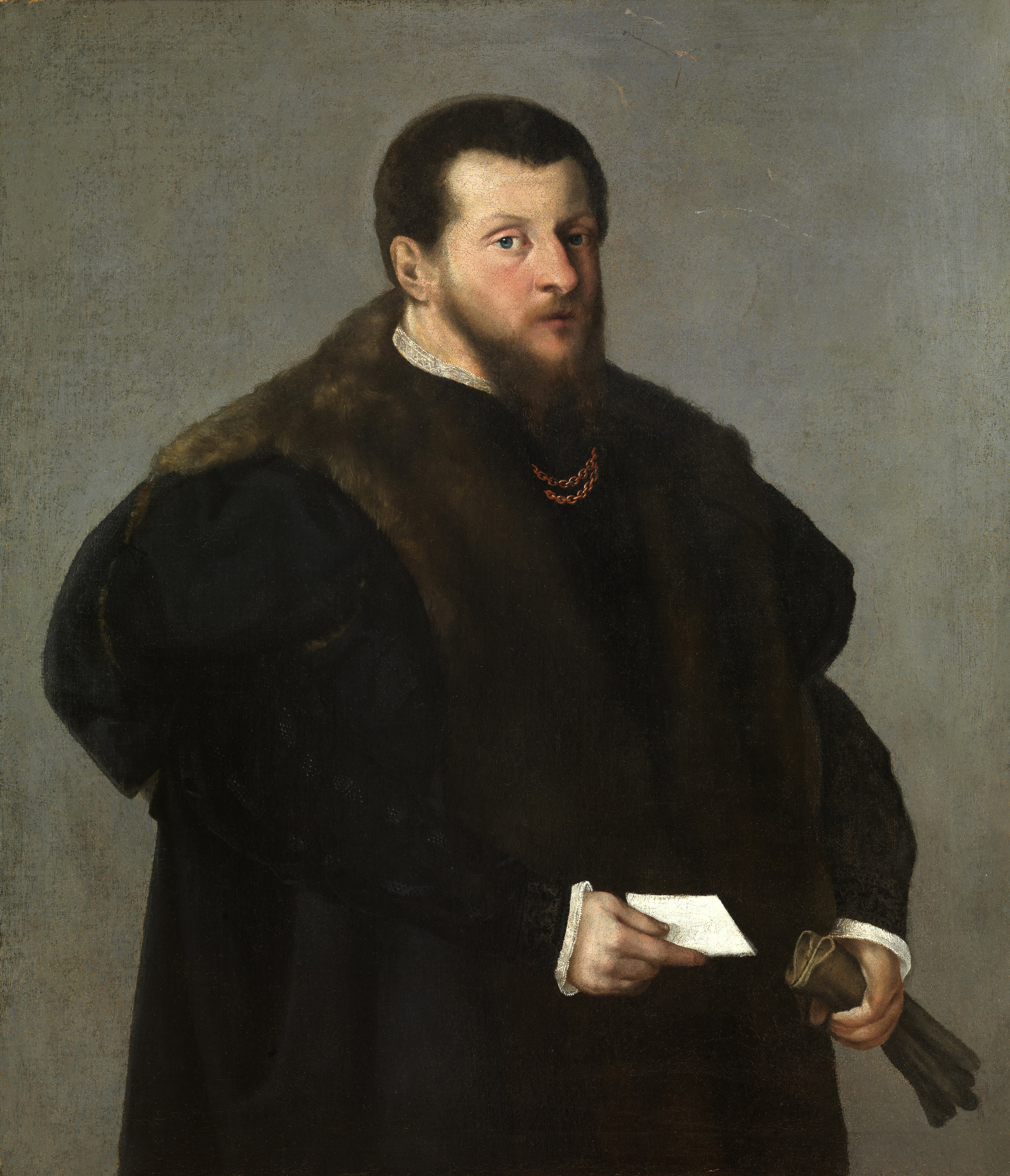The painting depicts a man from the 1600s or 1700s wearing a voluminous coat that appears dark brown to black, with a prominent, dark brown fur collar that encircles his neck and extends down his front, depicted with remarkable realism. The man has short black hair, a round head, and a pronounced, fuzzy brown beard and mustache. His attire includes a black vest beneath the fur collar, revealing two gold chains partially hidden by the layers of fabric, and a white collar peeking out underneath. He is looking straight ahead, making eye contact with the viewer. His left hand holds some kind of gray parchment or cloth, while his right hand grasps a white card. The overall impression is of a very wide torso, which could either be due to the man's robust build or the voluminous nature of his garments, which include large, dark, poofy sleeves.